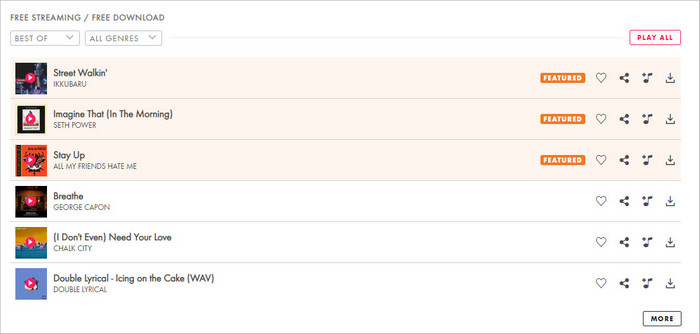The image depicts a sleek, modern app interface that appears to be a music streaming and downloading platform. The layout is approximately one and a half to twice as wide as it is tall, bordered by a thin black line. The primary background color is white.

In the upper left corner, the app prominently displays a notification: "Free Streaming / Free Download." Below this message, two small, rectangular drop-down boxes are positioned. The first drop-down box is labeled "Best Of" with a down arrow, and the second is labeled "All Genres," also with a down arrow. A horizontal gray line extends to the right of these elements. Additionally, there is a red-outlined button featuring red text that reads "Play All."

Beneath these controls, the interface showcases six distinct options, which appear to be either albums or songs. Each option is presented with an album cover on the left, adorned with a pink play button in the center. Accompanying these images, text labels specify the titles of each selection:

1. "Street Walking"
2. "Imagine That (In The Morning)"
3. "Stay Up"
4. "Breathe"
5. "(I Don't Even) Need Your Love"
6. "Double Lyrical - Icing on the Cake (WAV)"

To the right of each title, the interface includes a row of icons for different actions: a like button, a share button, a music note (whose function is unclear), and a download icon, enabling users to interact with each track.

Overall, the app interface is thoughtfully designed with a user-friendly arrangement, facilitating easy navigation and interaction within the music platform.